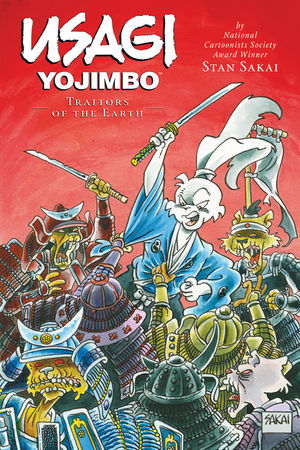This vertically aligned rectangular image appears to be the cover of a comic book. The upper portion features a bold red background with large white text in the upper left corner reading "USAGI YOJIMBO," with smaller tan-colored text beneath it that says "Traitors of the Earth." In the upper right corner, there's smaller white text stating, "By National Cartoonist Society Award winner Stan Sakai."

The lower portion of the cover is bustling with activity. At the center of the scene stands a prominent figure resembling a white rabbit, with its mouth wide open. This character is depicted wearing a blue robe with baggy sleeves and is holding a sword that boasts a gold handle and a silver tip. The rabbit's ears are bound together by a band, giving it a distinct samurai appearance. Surrounding this central figure are various creatures, including vampire-like rats and beings that have a mix of human and animalistic features. Some of these creatures wear armor and helmets adorned with horns, and all appear to be holding weapons, contributing to the chaotic and intense atmosphere. The background of the lower part of the image includes additional red hues that blend with the dynamic and busy scene below.